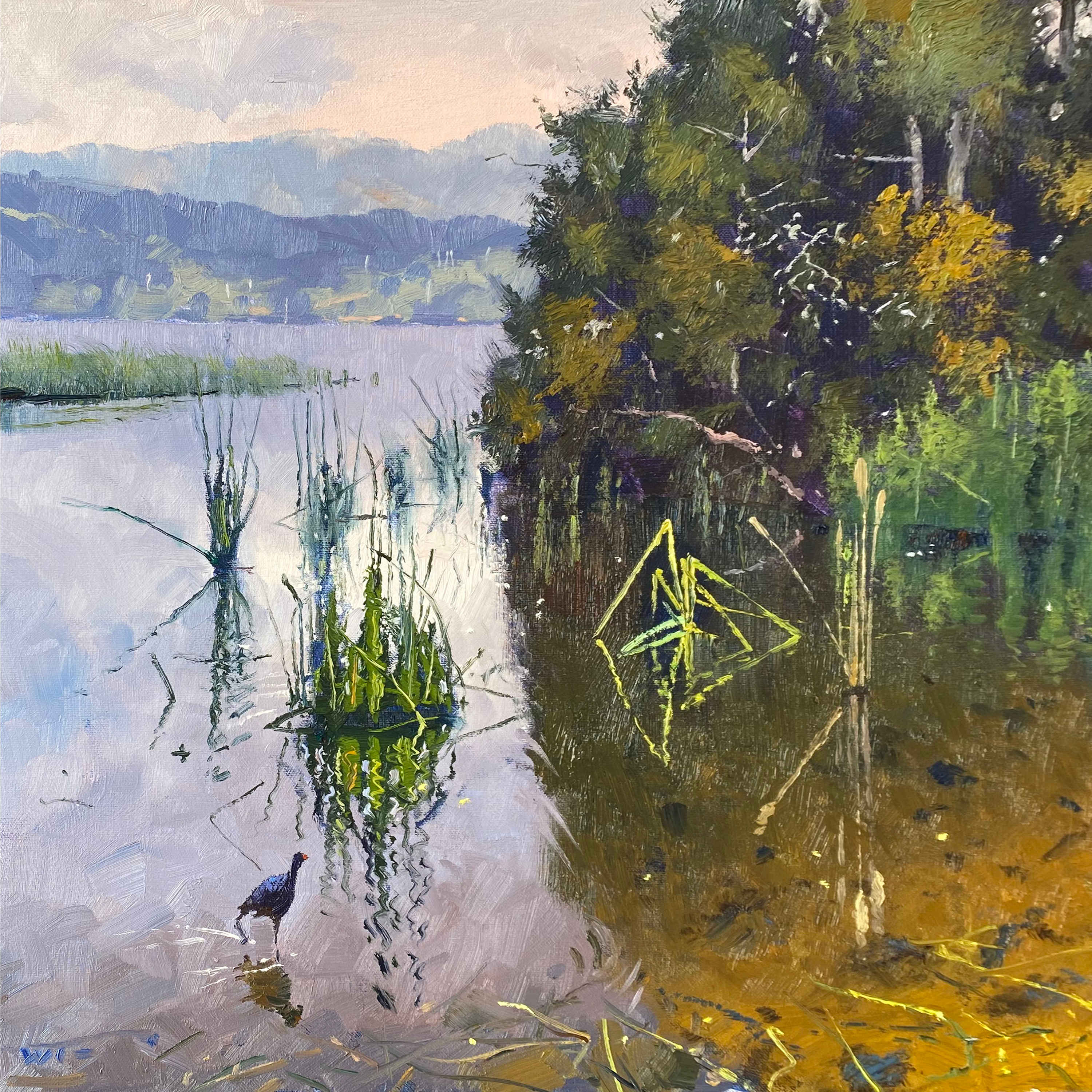This detailed painting depicts a serene, shallow body of water, likely a lake or swamp, characterized by its brown, muddy tones. In the foreground, a dark, possibly black or dark blue bird stands in the shallow water in the lower left corner, surrounded by vibrant green grasses and fronds. These plants grow out of the water, adding bright and vivid contrasts to the scene. Towards the right, clusters of green and yellow-green trees or a copse extend to the water's edge. The scenery in the background is somewhat blurred, showcasing distant mountains or a dense congregation of trees under a dull, murky gray sky. The entire scene portrays a pristine and tranquil natural environment with no visible signs of human presence, emphasizing the untouched beauty of this water-bordered landscape.